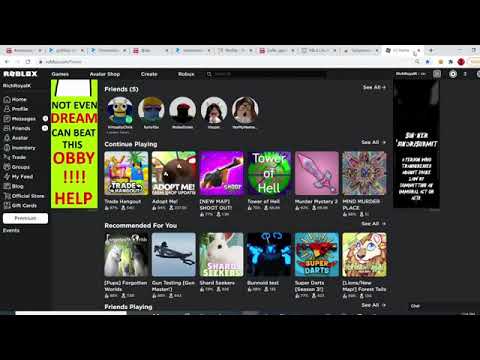This screenshot from Roblox features a top and bottom black border, each about an inch thick. The image is notably blurry. At the top beneath the black border, there's a gray toolbar with nine tabs, each containing an icon to the left and text to the right, though the blur prevents the details from being readable. Below this gray toolbar is a white strip holding a lengthy search bar. Continuing downward, the image transitions into another black section.

On the left side within this black section is a white "Roblox" logo, accompanied by indecipherable white text below it. Adjacent to this, there are approximately twelve small icons, followed by additional obscure white text and a clickable white tab marked by illegible black lettering. On the upper right, the words "Games," "Shop," and two other unreadable titles are visible.

Beneath "Games," a long lime green rectangle stands out. This rectangle features a white square at the top and several phrases in varying colors: "NOT EVEN" in black, "DREAM" in red, and "CAN BEAT THIS" in black followed by "OB" in red, punctuated by four exclamation points, and possibly the word "HELP."

To the left, a "Friends" section displays five profile pictures with names that are too blurry to distinguish. Below this, the image indicates a "Continue Playing" section with six game thumbnails, each accompanied by illegible game information. Further down, the caption "Recommended For You" appears in white text above another set of six game thumbnails.